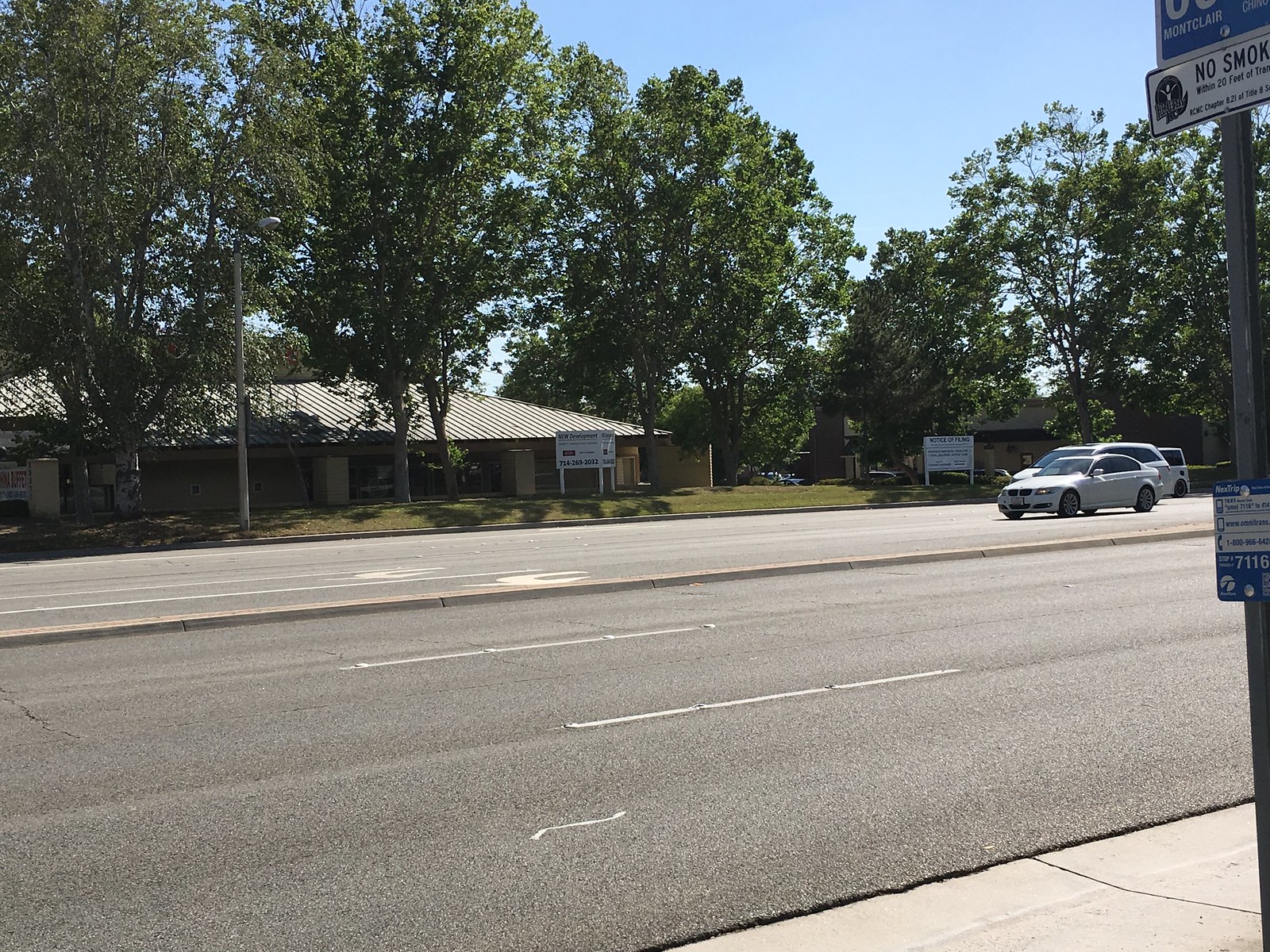The image captures a bustling multi-lane roadway as seen from a sidewalk perspective. A concrete divider splits the roads, providing a visual and physical barrier. The road to the right features two clearly marked left-turn lanes, evident by the arrows painted on the asphalt. On this road, two white cars are proceeding steadily forward. Towards the far right edge of the image, a signpost with multiple signs stands just out of frame, with one discernible sign indicating a no smoking zone on a white background.

Adjacent to the roadway, a small grassy median provides a natural buffer before transitioning to an architectural structure. This building stands with a brick foundation and a sloped metal roof, surrounded by a cluster of trees. Further detailing enhances the scene as several white signs emerge from the ground around the building’s perimeter. The road’s surface is characterized by numerous short white markings that guide the flow of traffic, contributing to the organized yet active atmosphere of the scene.